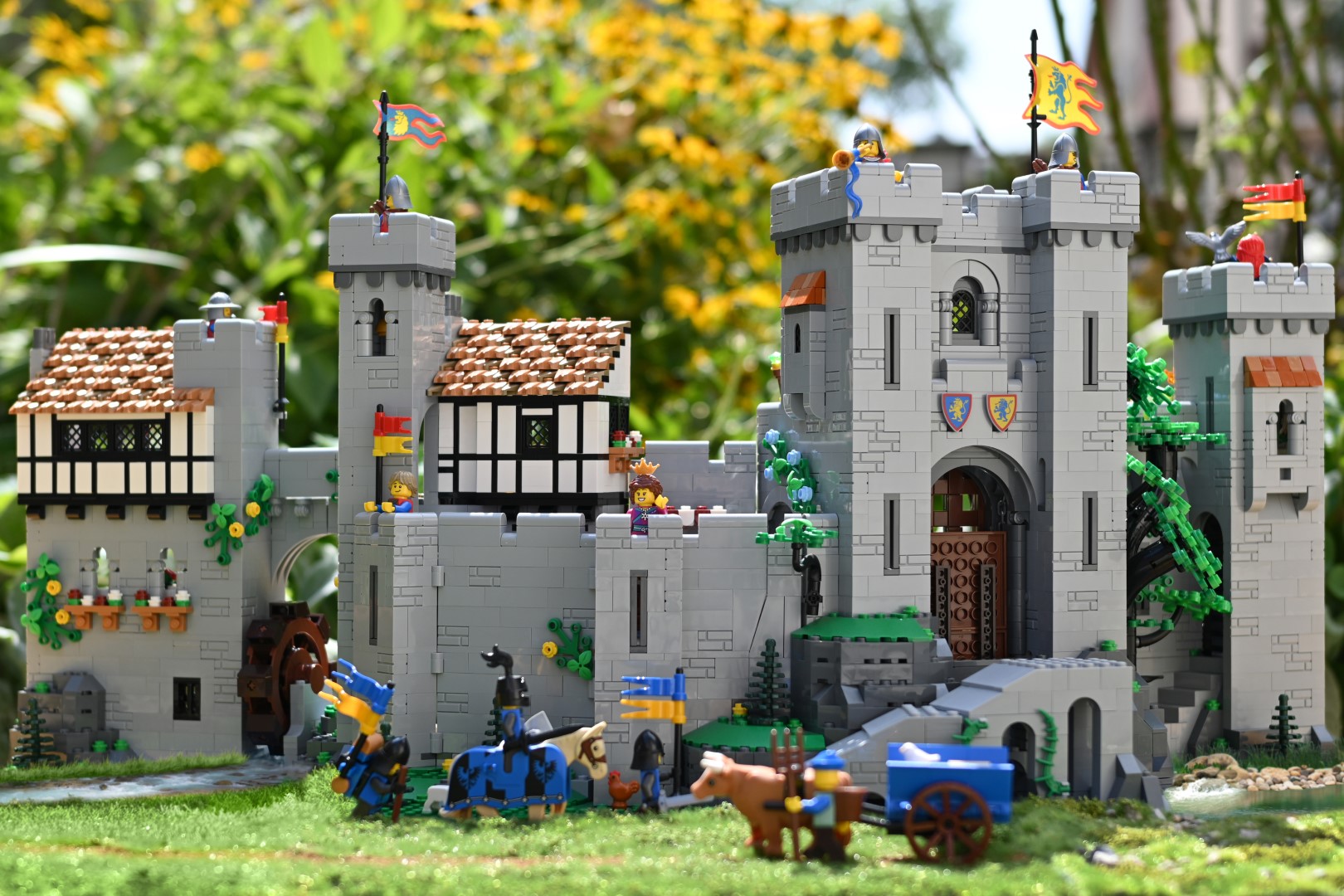The image depicts a detailed Lego castle scene set outdoors in a sunny environment. The rectangular photograph, wider than it is tall, showcases a large gray castle complete with four or five turrets, each adorned with red and yellow flags. Some of these flags depict animals, adding an extra layer of detail. Attached to the castle walls are flat-roofed towers and cream-colored awnings on the left side.

In front of the castle, Lego figurines are engaged in various activities: a knight on horseback, an oxen pulling a blue cart, and several other characters contributing to the village-like atmosphere. The scene is peppered with Lego elements such as greenery and flowers, enhancing the realistic touch.

The background reveals a juxtaposition between the Lego creation and the real world, with live grass, bushes, and trees that are somewhat faded, and a cream-colored house visible to the right. The photograph captures the intricately built Lego display vividly, with the outdoor natural setting making the castle blend seamlessly with what surrounds it.